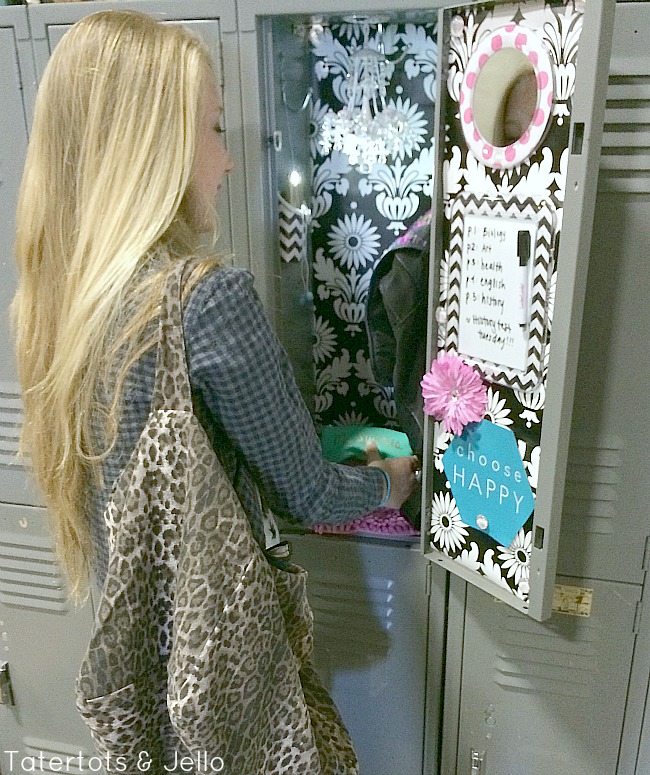This detailed photograph captures a young blonde girl, viewed from behind, as she organizes her well-decorated locker in a high school hallway. She is wearing a blue and black checkered long-sleeved shirt and has a leopard-print handbag slung over her right shoulder. Her long, straight blonde hair cascades to her waist. Inside her gray locker, adorned with intricate black and white floral and squiggly line patterns, several decorative items are noticeable. The locker door features a circular mirror framed with a white rim and dotted with pink polka dots. Just below the mirror, a flower decoration is affixed. A whiteboard with a black marker hangs centrally, next to a turquoise hexagon inscribed with the uplifting message, "Choose Happy," in white text. A mini chandelier and faux candles further embellish the vibrant space. The girl appears to be adjusting or placing a turquoise item inside the locker, which contains neatly arranged belongings. The overall scene is accentuated by white text in the bottom left corner of the image reading "Tater Tots and Jello".